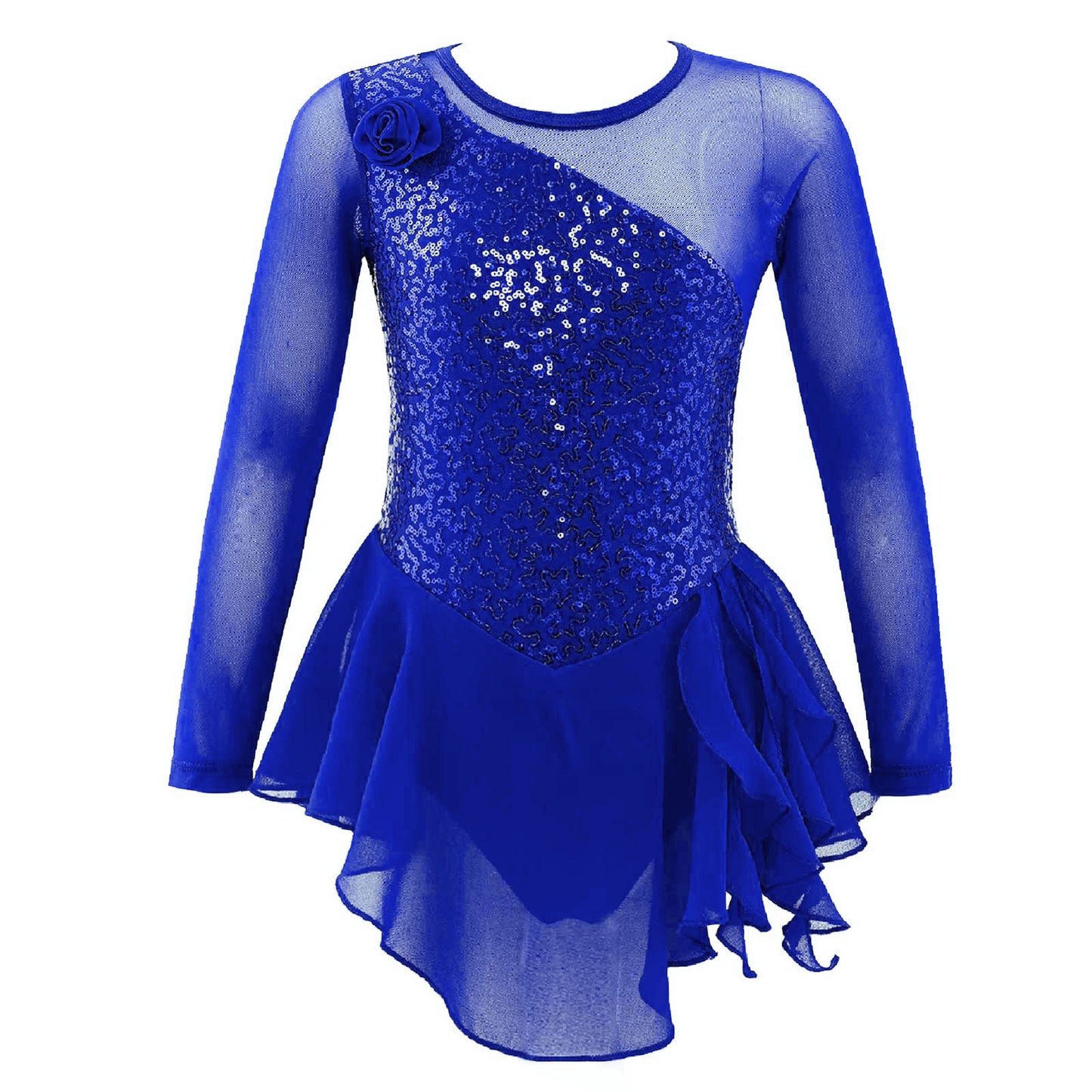This is a detailed, close-up photograph of a cobalt blue dance costume, likely designed for ballet or ice skating, set against a plain white background, giving it the appearance of floating in white space. The costume resembles a one-piece leotard with an attached frilly tutu skirt. The upper portion features sheer, almost opaque long sleeves that allow a glimpse of skin beneath, giving an elegant and delicate look. Draping diagonally across the chest is a sparkly overlay made from small, shimmering discs, tapering down the torso and interspersed with silver, white, and black rhinestones. A striking blue rose corsage adorns the left shoulder, just before the sheer material meets the sequined section, adding a touch of sophistication. The seamless blend of fabric and intricate detailing makes it appear as if it's modeled on a mannequin, edited to enhance focus purely on the garment, akin to a high-quality e-commerce presentation.